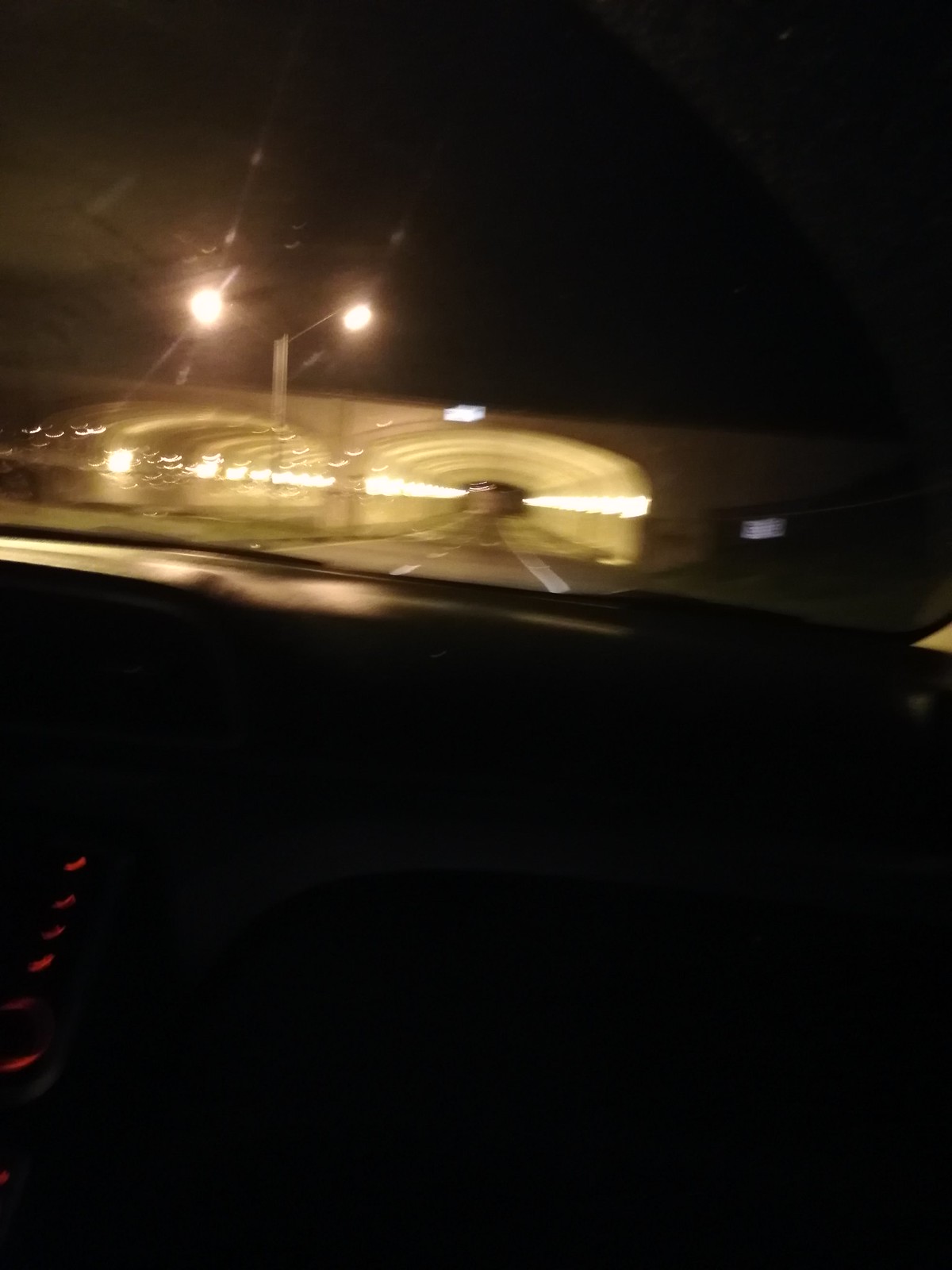A night-time scene capturing a vehicle approaching the entrance of a tunnel. The darkness is pierced by an array of bright reflections, indicative of the late hour. Streetlights and headlights cast an intricate web of light and shadow across the road. A distinct laser-like beam extends horizontally from left to right, interrupted only by the tunnel's opening. Additional overhead lights guide drivers into the tunnel. The clear, dry pavement hints at a crisp, clear night, enhancing the eerie, almost haunting atmosphere of the image.